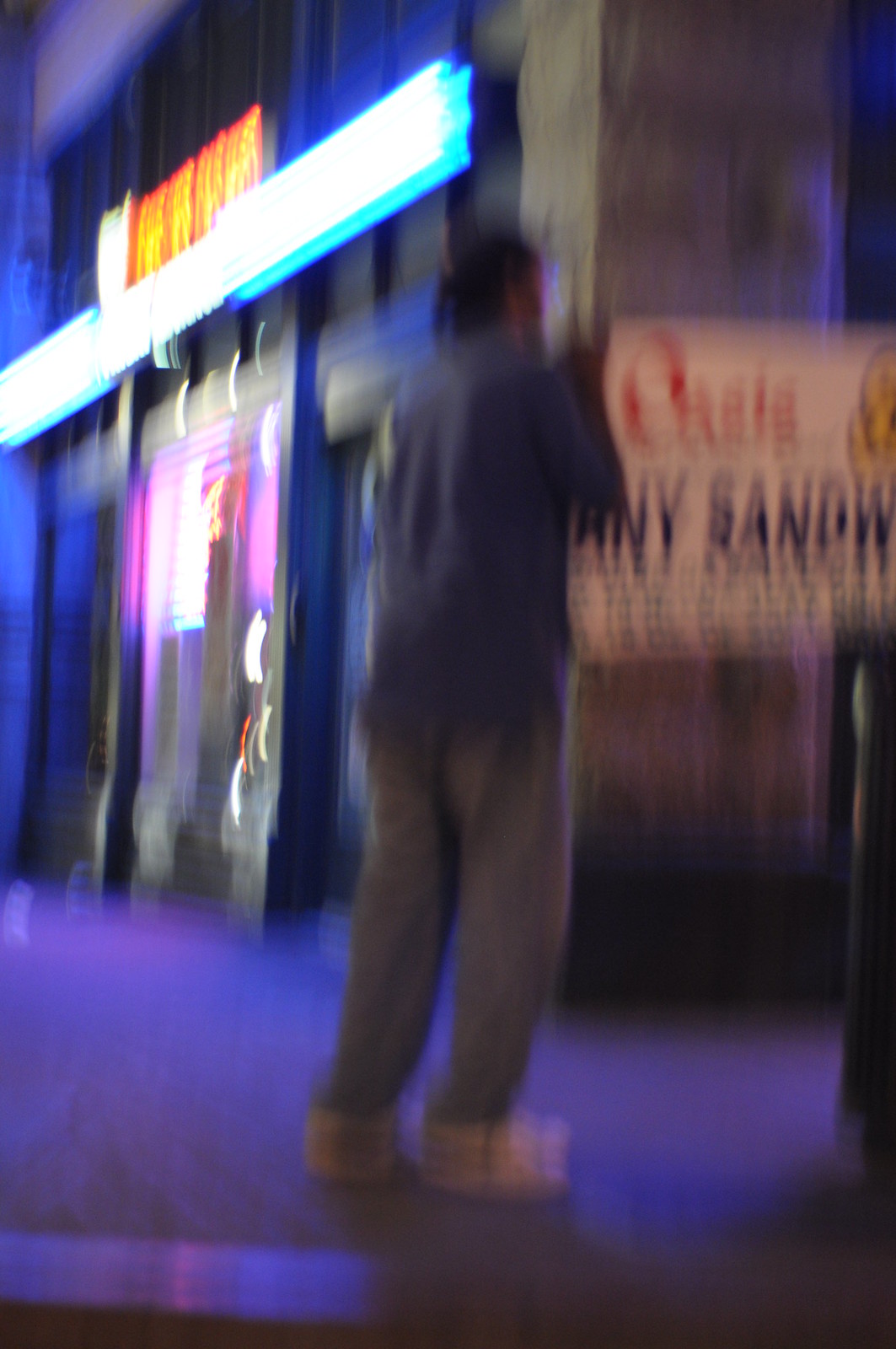A blurry nighttime photograph captures the back of a person standing in the center of the frame, seemingly a man with dark hair possibly pulled into a ponytail. He wears a dark blue shirt, light blue or gray jeans, and white shoes. His skin appears fair, although details are hard to make out due to the blurriness. To his right, there is a large, possibly stone or cinder block pillar at the corner of a building. Behind him, a white sign with red lettering partially reads "Any [Sandwich]," while a larger sign with "Oasis" in red and another unreadable phrase in dark blue or black lettering is visible. Above the pillar, a rectangular neon sign emits a bright blue light, with an orange sign above it, casting a bluish-purple glow onto the surrounding sidewalk. The scene is dimly lit yet vibrant, with multiple neon and illuminated signs contributing to the atmosphere.